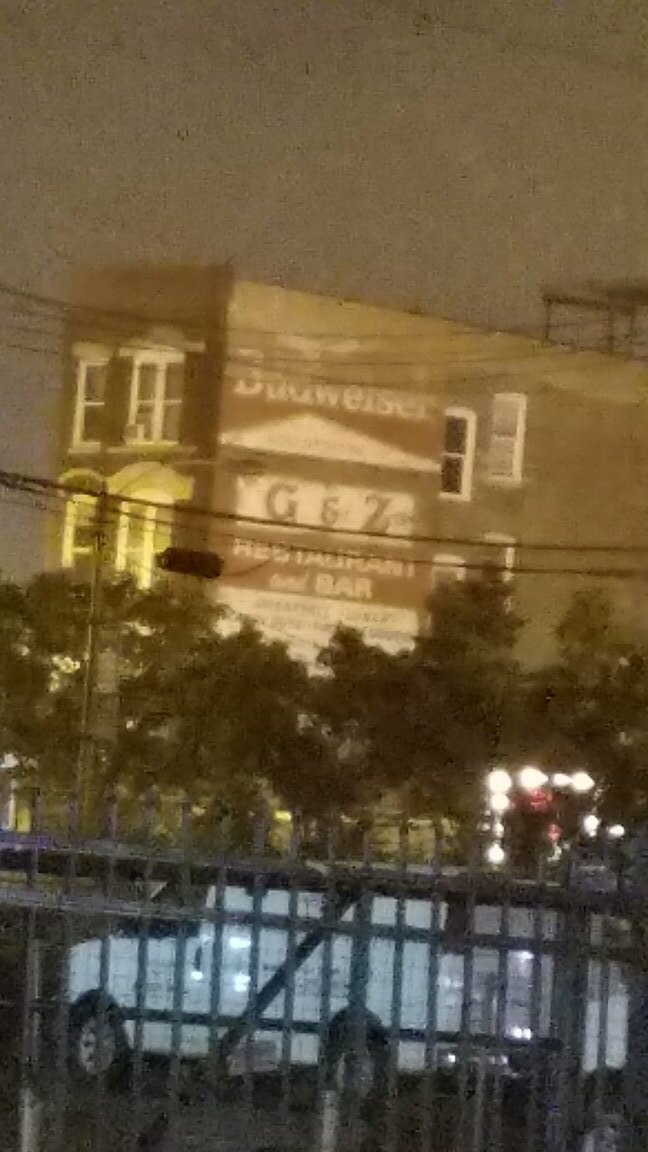This grainy, nighttime photograph captures an urban scene with various elements. Along the bottom of the image, there is a metal-barred fence, through which a white van with text on its side is visible, along with the front of another vehicle to its right. Both vehicles are facing left, suggesting they are parked or moving in that direction. Behind the vehicles, there's a row of trees spanning across the image from left to right, interspersed with telephone or electrical poles and wires. In the background, a large, dark brown factory-like building is prominent, with the word "Budweiser" clearly displayed on it. The building features various geometric shapes and appears to be at least two to three stories tall. Despite the dark setting and pixelation, distinctive details like small black specks and squiggly lines are noticeable on the image, contributing to its overall graininess.